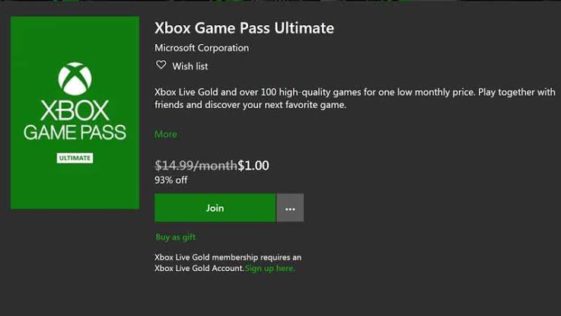**Detailed Caption:**

This image is a screenshot featuring an advertisement banner for Xbox Game Pass Ultimate. The overall design of the banner is set against a very dark background, ranging from nearly black to deep gray tones. On the left side, there is a prominent, tall green triangle that includes the Xbox Game Pass logo along with the Xbox emblem. At the lower part of the triangle, a white button labeled "Ultimate" is visible, emphasizing the product name.

Adjacent to this green triangle, the dark background continues to the right, creating a contrast that makes the text and buttons stand out. At the top of the banner, the text reads "Xbox Game Pass Ultimate" along with "Microsoft Corporation," followed by a clickable button that allows users to add the product to their wish list.

The advertisement highlights the features of Xbox Game Pass Ultimate: "Xbox Live Gold and over 100 high quality games for one low monthly price. Play together with friends and discover your next favorite game." Below this description, a green button with the word "More" appears.

The original price of the service, $14.99 per month, is shown but has been grayed out and crossed out. It is currently on sale for $1.00, representing a 93% discount. Under this promotional price, there is a green "Join" button for users interested in subscribing, followed by a link labeled "Buy as a Gift."

At the very bottom of the page, there is a note stating, "Xbox Live Gold Membership requires an Xbox Live Gold account. Sign up here."

Overall, the banner ad effectively uses color contrast and clear messaging to promote the Xbox Game Pass Ultimate service and its features.